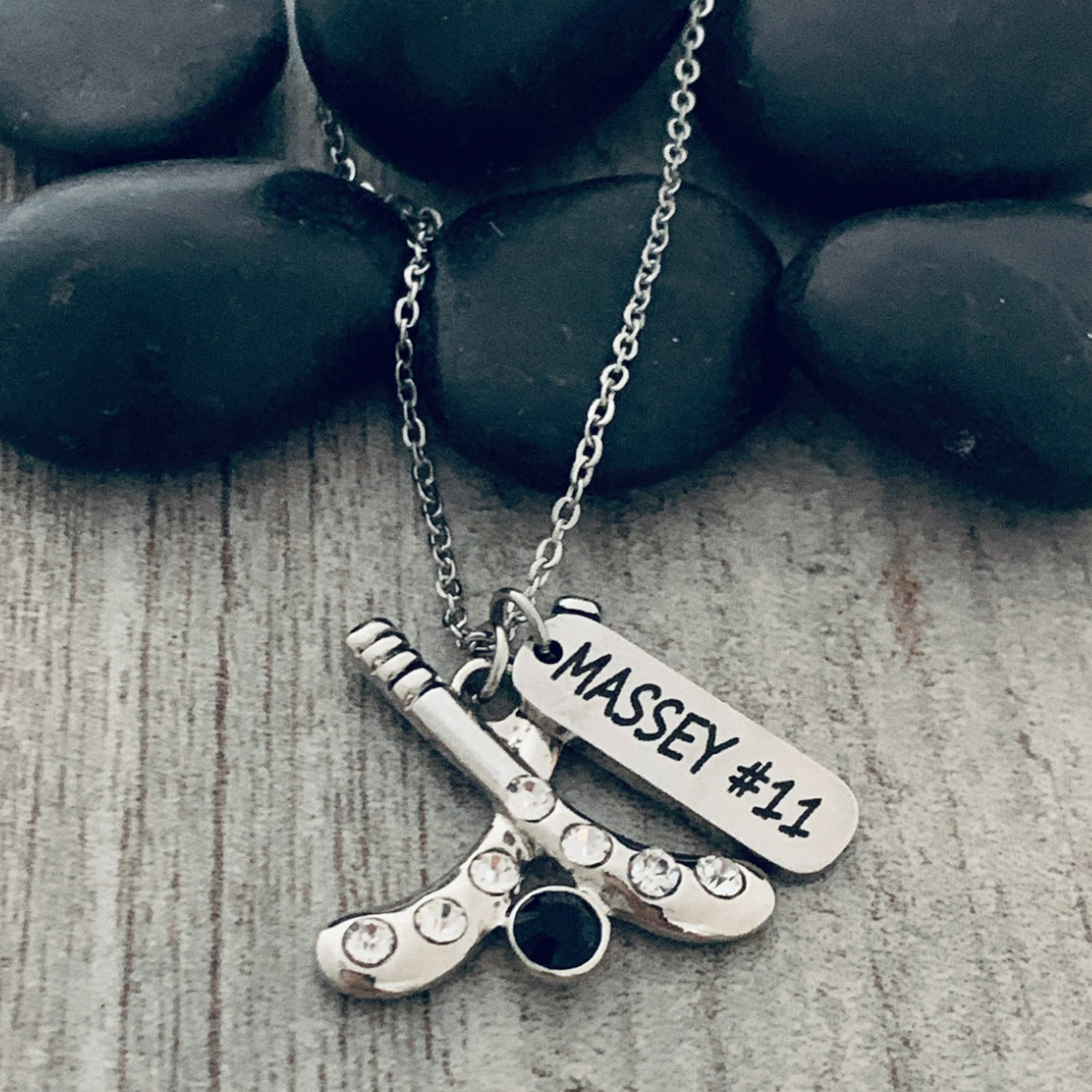This is a detailed photograph of a silver necklace resting on a gray, wood grain surface. The necklace features two notable charms: one is a long, slender dog tag inscribed with "Massey" and the number "11," and the other is a pair of hockey sticks crossed to form an X, with a hockey puck at the center and gemstones encrusted along the sticks' lengths. The silver chain of the necklace is artistically draped over six smooth, black river rocks positioned at the upper portion of the image. The careful arrangement and intricate details, such as the black font on the charms and the jewelled hockey sticks, suggest this piece of jewelry is specially designed, possibly commemorating a player named Massey associated with the number 11.